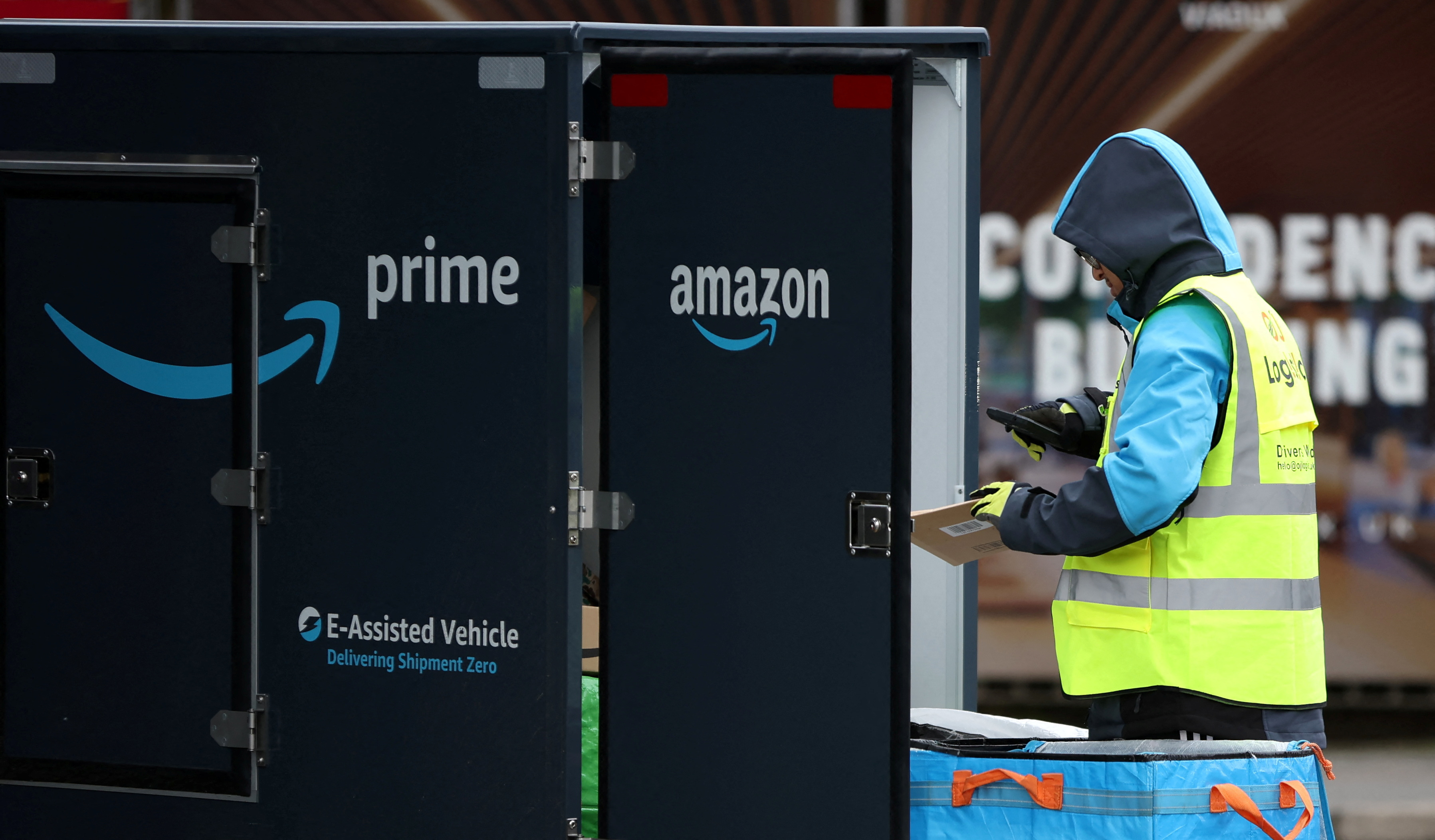In this horizontally rectangular exterior shot, the left side of the frame prominently features the back end of an Amazon delivery vehicle. The back door of the vehicle is open, revealing the "Prime" logo on the side of the truck and the "Amazon" logo on the door. At the bottom of the side panel, it reads, "E-Assisted Vehicle, Delivering Shipment Zero". On the right side of the frame, a person in a black and teal hoodie with a yellow hazard vest is visible, looking down at some equipment in their right hand, which appears to be a scanner. In their left hand, beneath the scanner, they hold a package resembling a manila envelope. The individual’s face is not visible, making it difficult to determine their identity or gender. In the foreground, at the bottom of the frame, there is a large light blue bin with bright orange handles, likely used for carrying packages.